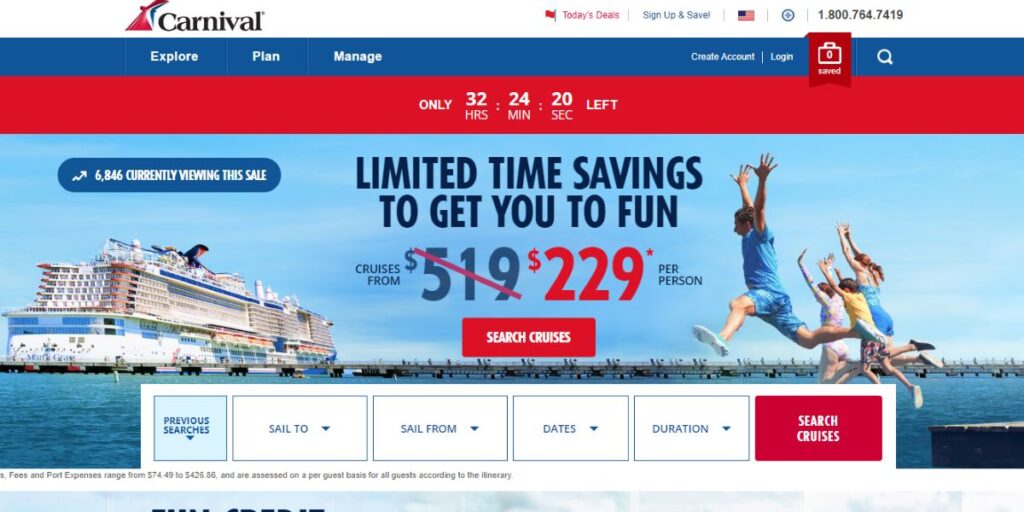At first glance, the image appears to be a screenshot of the webpage for Carnival Cruise Lines, a prominent cruise ship company. Positioned at the top left is the recognizable Carnival logo, while the top right section features text in multiple colors: "Today's Deals" in red, "Sign up and save" in black, an American flag icon, a plus sign, and their contact number, 1-800-764-7419.

The background of the webpage features a combination of dark blue, red, and light blue hues. Spanning the top of the page from left to right are several navigation tabs: "Explore," "Plan," "Manage," "Create Account/Log In," "Saved," and a magnifying glass icon for search functionality.

Directly beneath these tabs, on a prominent red bar, there is a timer counting down with the text "Only 32 hours, 24 minutes, and 20 seconds left." Below the timer, the left side of the page showcases an image of a grand cruise ship sailing on blue waters against a backdrop of a clear blue sky. To the right, there's an image of a family, seemingly jumping off a pier into the water, but upon closer inspection, it appears to be a Photoshop edit as they are not dressed in swimsuits. The family consists of a mother, father, and two children. The parents are dressed in blue attire, while one child wears a yellow shirt and the other a white shirt. The portrayal suggests they are jumping in excitement rather than into the water.

On the left, within a small blue oval, there's text indicating "6,846 currently viewing this sale." The central section provides details about the promotional offer: "Limited time savings to get you to fun. Cruises from $519," with the original price crossed out and the discounted rate of $229 per person highlighted in red. Adjacent to this is a "Search Cruises" prompt.

Below, there are drop-down boxes for refining search criteria: "Previous searches," "Sail to," "Sail from," "Dates," and "Duration." A prominent red "Search Cruises" button is also visible. Additionally, there's a note detailing fees: "Fees and Port Expenses range from $74.49 to $426.86 and are assessed on a per-guest basis for all guests according to the itinerary."

In summary, this is the Carnival Cruise Lines webpage presenting a time-limited sale with substantial savings and detailed navigation options for potential bookers.